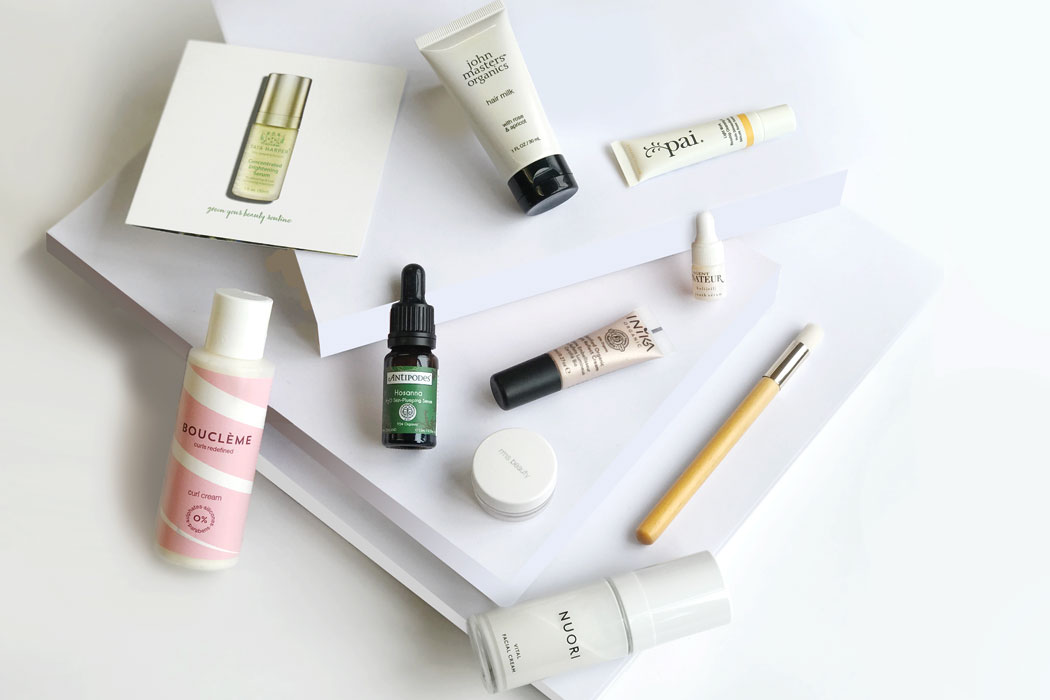The image shows an aerial view of several beauty products arranged on white shelving units. On the left, there is a small bottle of lotion labeled "SOUCLENE" with a pink and white design. Next to it, to the right, is a tiny green dropper bottle with a black dropper. In front of this is a small, flat white jar. Behind the jar, there's a gold-colored tube with black text and a black cap. Farther right, there's another small white dropper bottle.

On the shelf below, a makeup brush lies next to a white bottle labeled "NUORI." Above this, there's a container labeled "John Masters Organics" with a black lid, designed for squeezing out the product. To its right, there's another lotion container labeled "PAI." To the far left, there appears to be a piece of white paper displaying an image of a yellow bottle with green text and a gold lid.